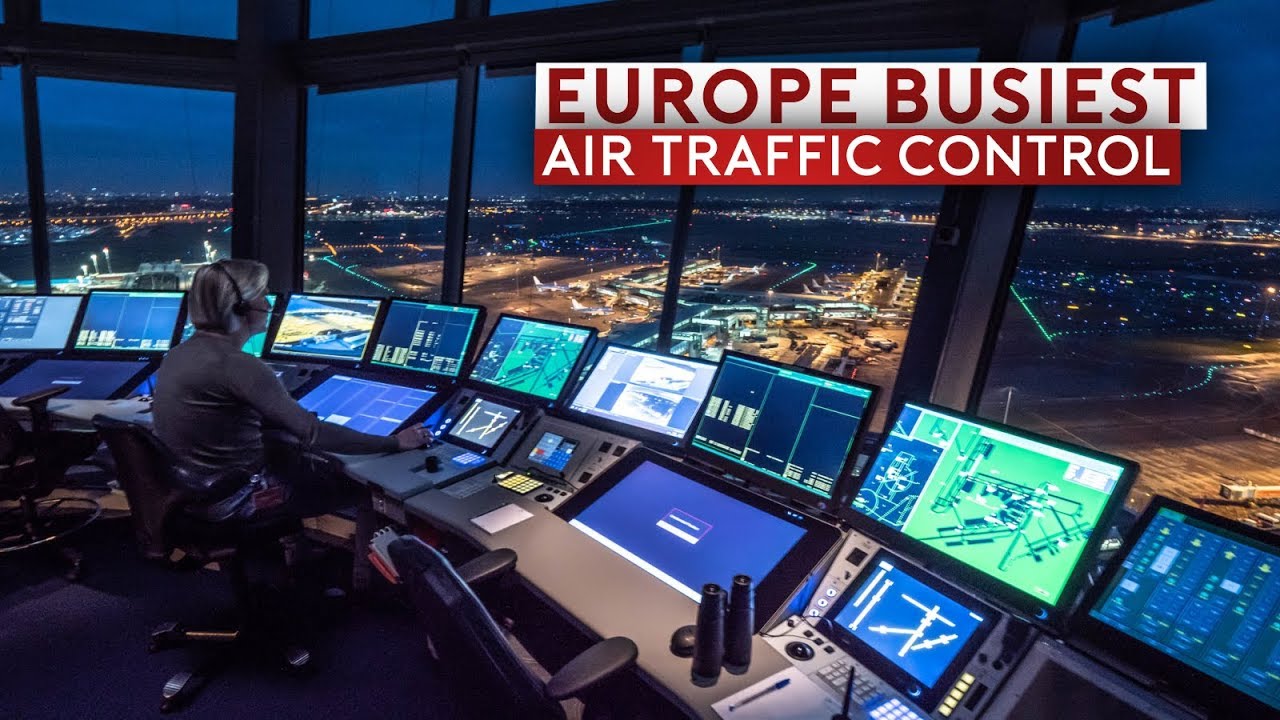The image captures Europe's busiest air traffic control tower, framed by a distinctive alternating white and red border—white at the top right and red below—with the text 'Europe's Busiest' in red font on a white background and 'Air Traffic Control' in white font on a red background. Within the tower, a single air traffic controller with silver hair, wearing a grey long sleeve shirt and blue jeans, sits at a desk heavy with technology. Two rows of multiple computer screens, displaying a mix of blue and green text and images, dominate the control panel. Essentials like a headset, binoculars, a pen, and a pad are strategically placed on the desk amid three desk chairs. The scene outside the large, wall-spanning windows reveals an airfield speckled with green dotted runway lights and a variety of planes, set against the backdrop of a dark blue sky indicating early evening or pre-dawn. The distant city skyline, lit up with buildings and homes, adds depth to the panoramic view.